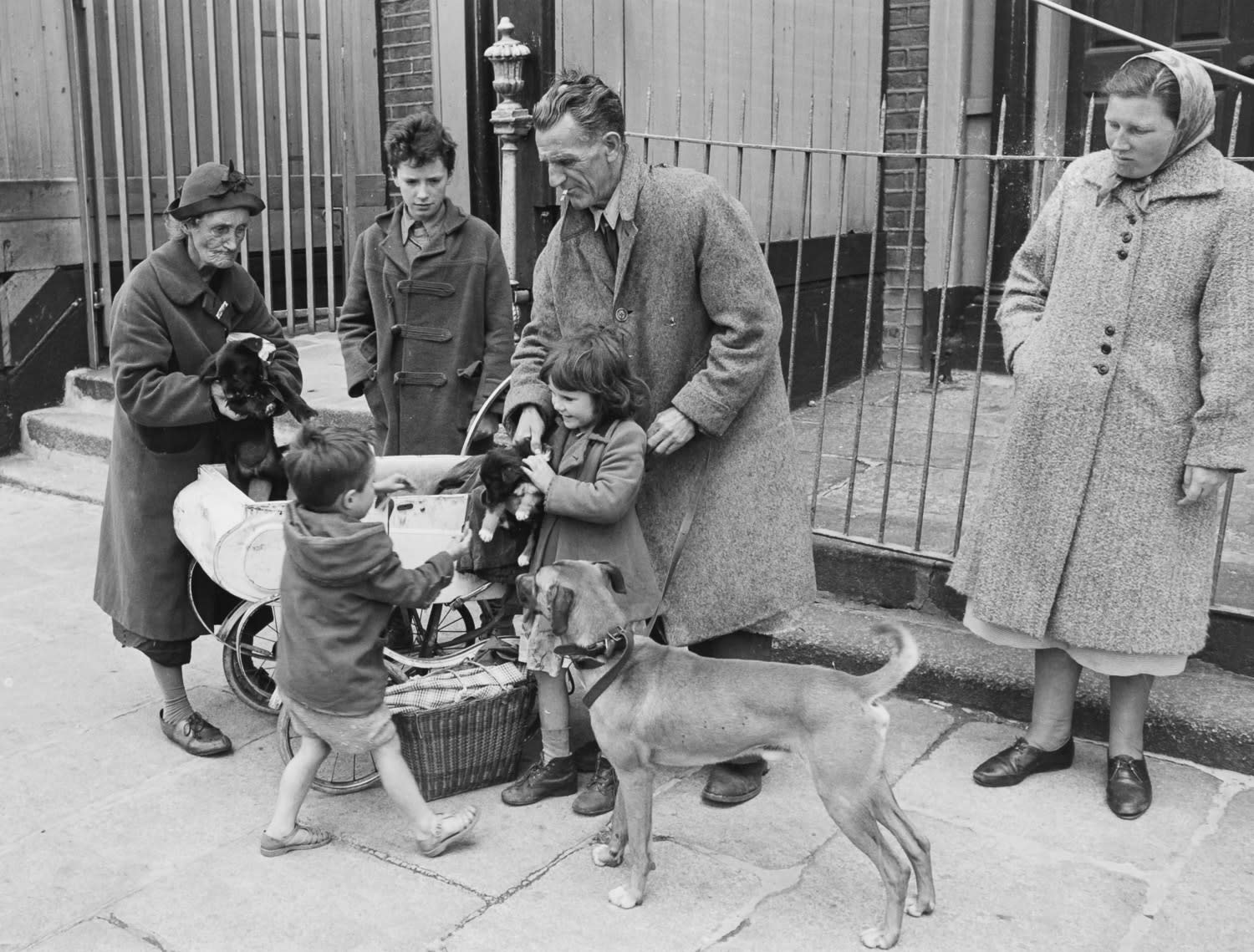This rectangular black and white photograph, wider than it is tall, captures an urban sidewalk scene during the day. The photo, likely old given its monochromatic tone, features a group of people clad in winter coats. At the center stands a man in a heavy gray overcoat, holding a dog's leash. The dog, a medium-sized breed, is attentively looking at the children. In front of the man is a young girl, around six or seven years old, wearing a similar coat, and in front of her is a slightly younger boy, possibly five years old. To the man's right, there is a middle-aged woman in a long gray coat and dress, her head partially covered, who is looking down towards the children. On the far left stands an older lady in a dark gray coat and hat, also observing the scene. Completing the group are two other adults in gray coats, positioned near a metal fence with additional metal slabs extending up to the left-hand corner of the photo. A classic baby stroller and a basket are placed on the ground behind the children, while the sidewalk beneath them is composed of large concrete squares. The image conveys a moment of interaction among the people, framed by the surrounding urban landscape.